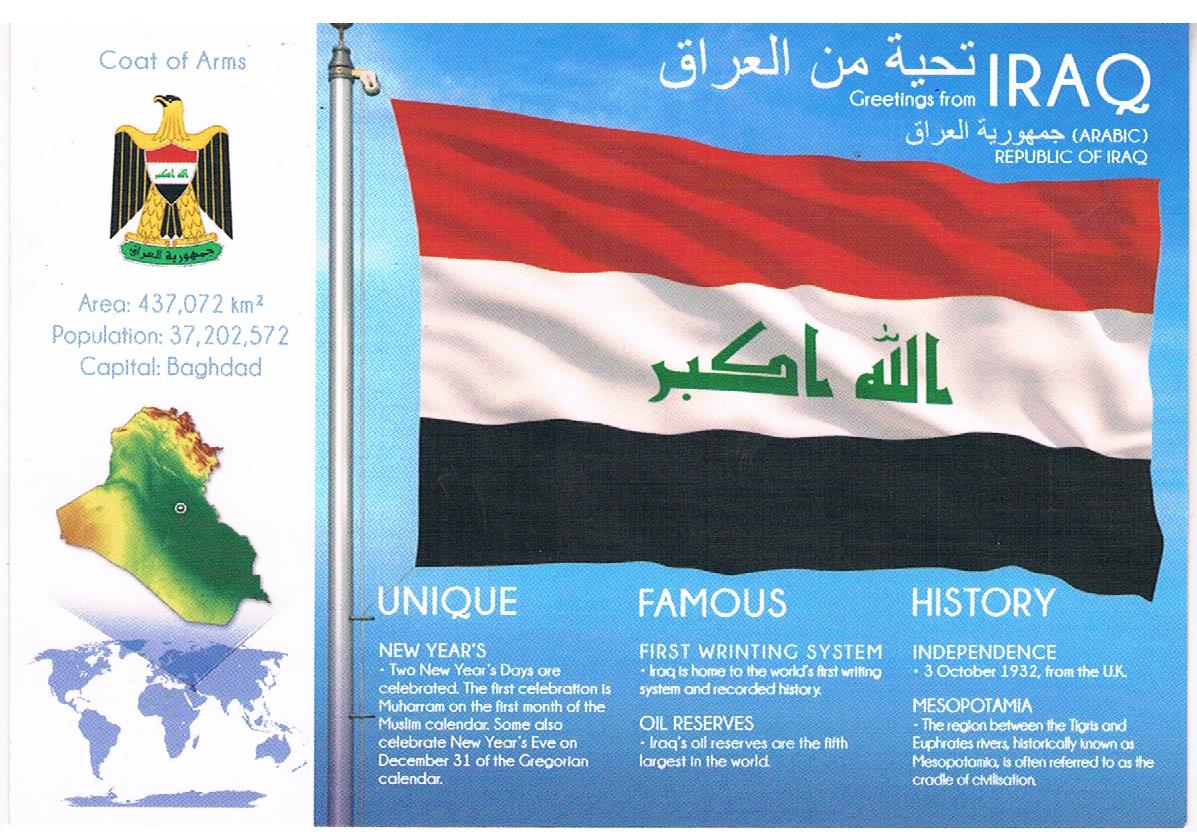A computer-generated image depicts the Iraqi flag waving gracefully from a flagpole against a serene backdrop of blue skies. The flag, centered and facing towards the right, showcases the traditional colors of black, white, red, and green. Prominently, white Arabic script adorns the central white stripe, flanked by red and black bands above and below respectively. The flag's intricate detailing includes a map of Iraq and the symbolic Golden Eagle or Falcon, highlighted within the design. Beneath the flag, the word "Iraq" is inscribed in English, emphasizing the nation's unique and storied history. This depiction, with elements hinting at Iraq's New Year celebrations, the pioneering first writing system, its journey to independence, and rich oil reserves, artistically merges historical significance with contemporary digital artistry.